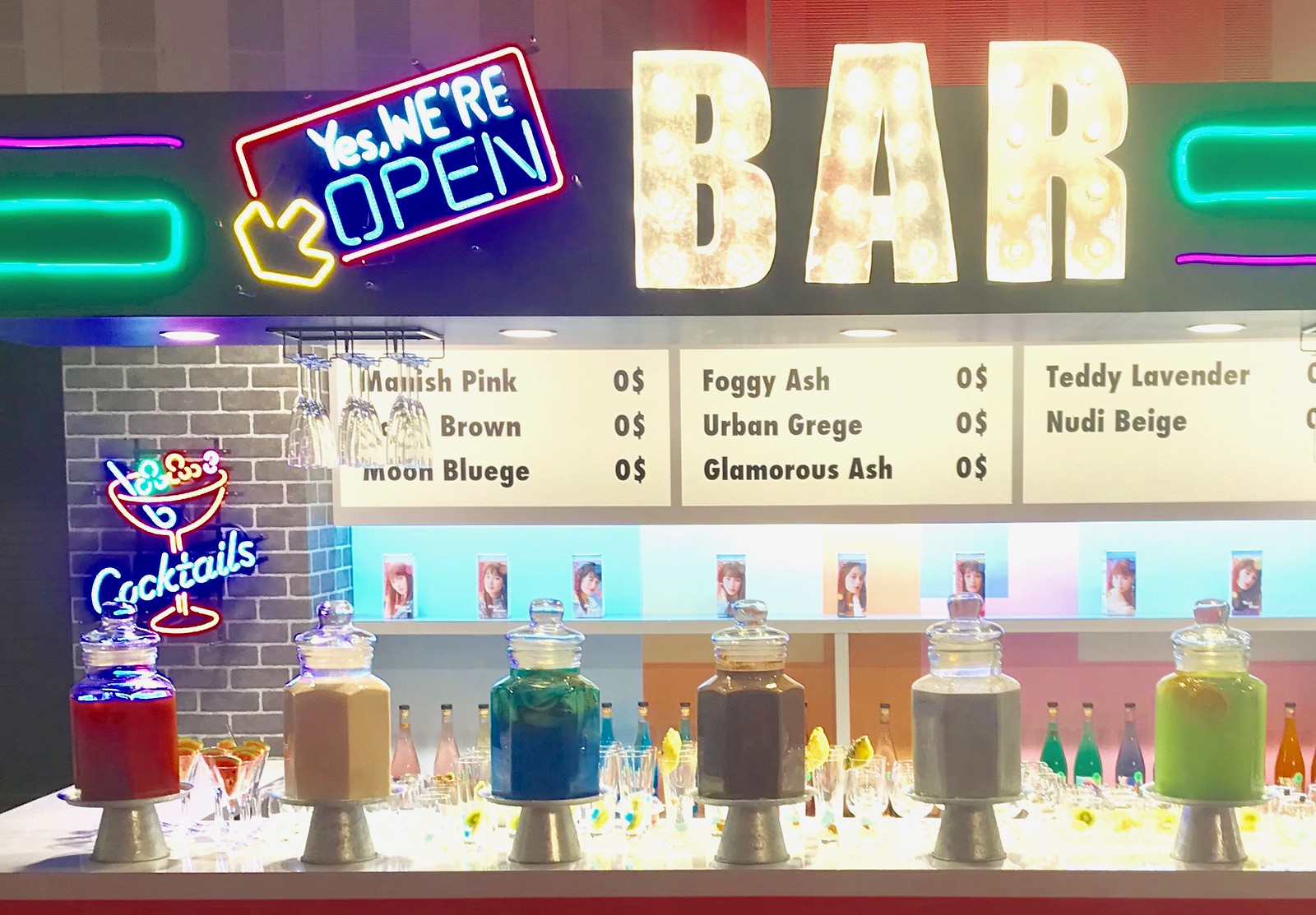The photograph showcases a vibrant cocktail bar with a lively atmosphere, featuring colorful neon signs and eye-catching details. At the top, prominently displayed in big, bright white letters, is the word "BAR" illuminated with a neon glow. To the left, a neon sign reads "Yes, we are open," with a yellow arrow pointing down towards the bar area. Directly below the large "BAR" sign are three white boards with black lettering listing the names and prices of various drinks, such as Foggy Ash, Urban Greggé, Glamorous Ash, Teddy Lavender, and more.

A portion of the brick wall features a neon sign of a cocktail drink that reads "Cocktails," adding to the festive ambiance. In the foreground, a table is laden with glass bottles containing liquids of various vibrant colors: red, tan, blue, brown, gray, and green. Surrounding the bottles are numerous empty glasses, ready for serving. The menu board in the background details the available drinks and their prices, and photo frames featuring women's faces enhance the decor. The entire scene is set against the backdrop of what appears to be digital artwork, giving the impression of a video game promotion or a modern, stylized bar representation.